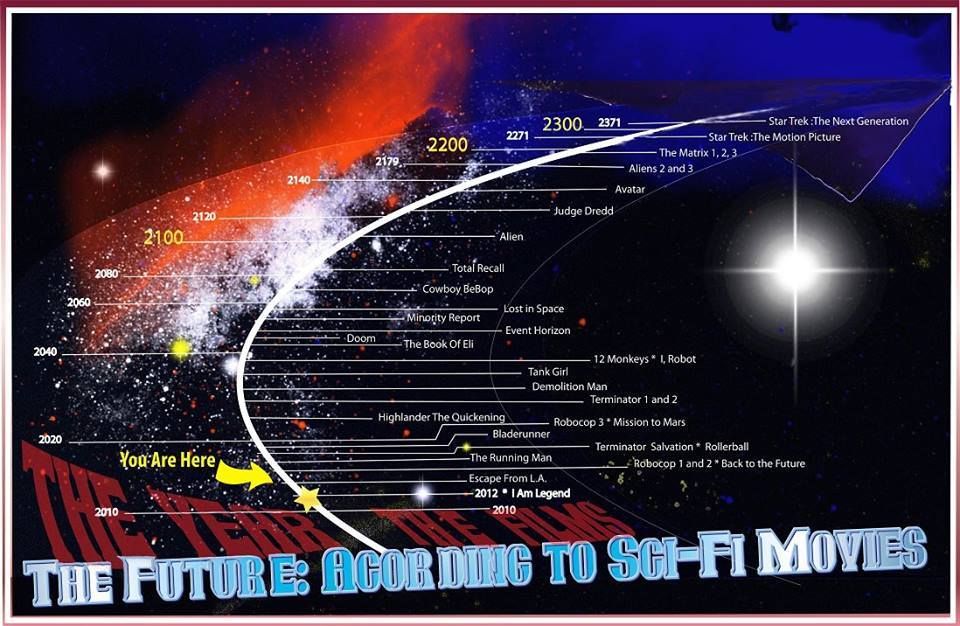The image is a rectangular graphic approximately six inches wide and three inches high, bordered with a thin maroon line at the top and bottom, with the sides fading to white. Within this border is a depiction of outer space, featuring a dark blue and black background, accented with a red band transitioning from the lower left to the upper right, and a bright white star on the right side.

The graphic serves as a timeline detailing future years as portrayed in sci-fi movies, with the title "The Future According to Sci-Fi Movies" in block blue print at the bottom right, and above it, in red print, "The Year, The Films." A curved white line extends diagonally, listing years from 2010 to beyond 2371, with corresponding films. 

A yellow banner with a star marks the current year, labeled "You Are Here" and "2012," alongside "I Am Legend." Films mapped out include "Escape from L.A.," "Robocop," "Back to the Future," "The Running Man," and "Terminator," among others, progressing through future years: "Robocop 3" (2020), "I, Robot" (2040), "Cowboy Bebop" (2071), "Total Recall" (2080), "Alien" (2100), "Dredd" and "Avatar" (2120), "The Matrix" series, "Star Trek" (2271), and "Star Trek: The Next Generation" (2371).